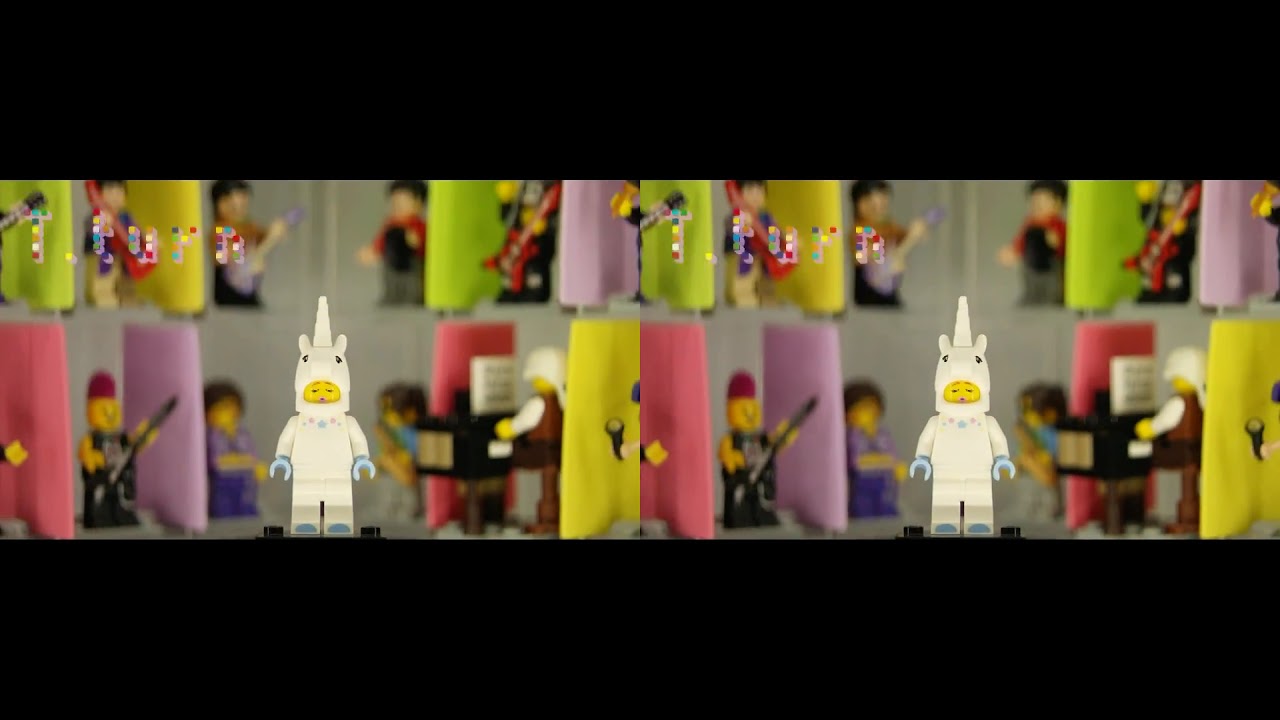The image is set within a horizontal rectangular frame, bordered by thick black bands on the top and bottom. Nestled at the center are two identical figures resembling Lego characters dressed in white unicorn costumes, complete with tall white horns and pale blue claw-like hands. Their facial features include yellow snouts and black eyes. The backdrop features an array of blurred, vibrant Lego pieces organized on shelves. The shelves display a mixture of multicolored tubes—green, yellow, pink, and purple—interspersed with various figurines. Among these, a Lego figure with red hair playing a guitar and another playing a piano stand out, although there are repeated figurines throughout the scene. Additionally, at the top of the image, pixelated multicolored text seems to spell out "T TURN" in two places, though the text remains somewhat ambiguous.